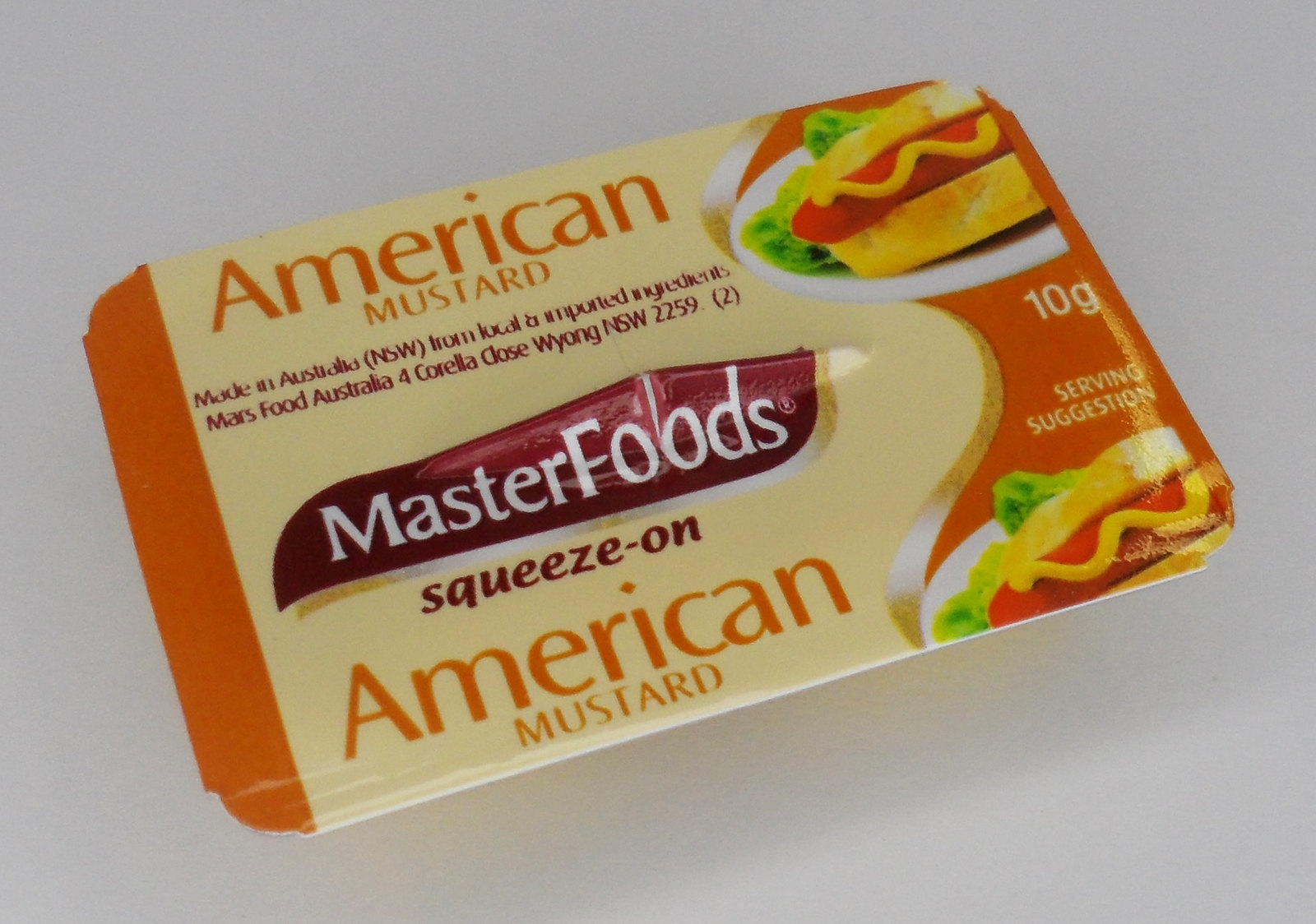The image displays a packet of American mustard, positioned at an angle. The packet features a peel-off top and prominently states "American Mustard" in bright orange font on a yellow background. Despite its name, the mustard is made in Australia by Mars Food Australia, as indicated by the text on the packet. The packaging includes the address "4 Corella Close, Wyong, NSW 2259" and mentions that the product is made from local and imported ingredients by the brand Master Foods.

On the left side of the packet, there is an orange stripe, while on the right side, there are two small, mirrored images of a sandwich which appears to be a hot dog with a smear of mustard down the middle, placed on a bed of lettuce. The text "squeeze on" and "American Mustard" is also printed on the packet. The mustard packet is 10 grams in weight, and the images serve as a possible serving suggestion.